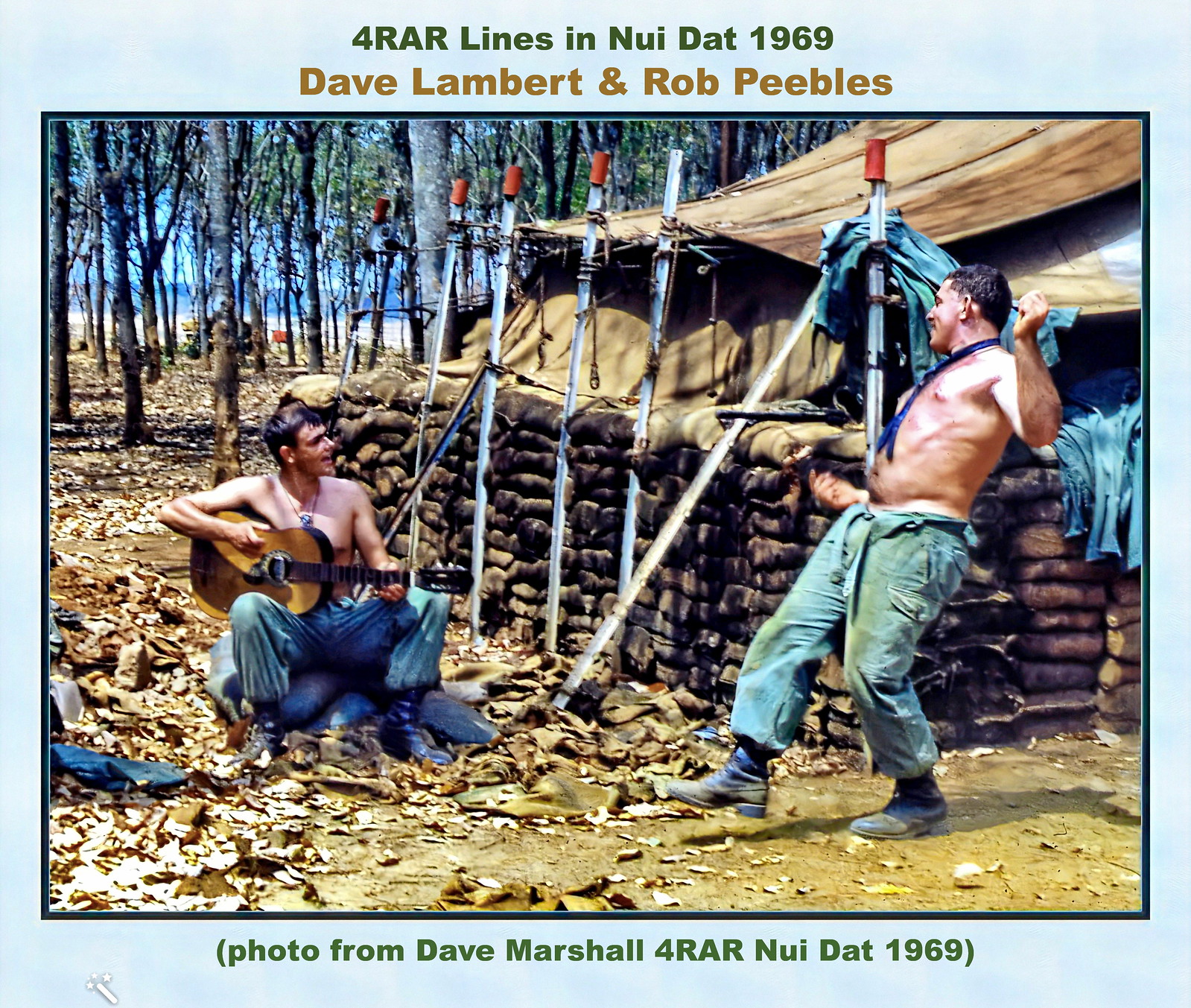The photograph features two shirtless men at a military camp in a lightly wooded area with sparse tree coverage. The camp includes a large canvas tent surrounded by piled sandbags. Both men, who are identified as Dave Lambert and Rob Peebles, are wearing military pants and boots. The man on the left, a white guy, is sitting down and playing the guitar, looking towards his companion. The other man is standing, leaning back as if dancing, with one arm bent upwards and the other arm down at his side, and appears to be wearing a blue necktie. The image has a light blue border. Above the photo, it reads "4 R.A.R. lines in N.U.I.D.A.T. 1969," and within the border beneath the photo, it says "Photo from Dave Marshall, 4 RAR N.U.I.D.A.T. 1969."